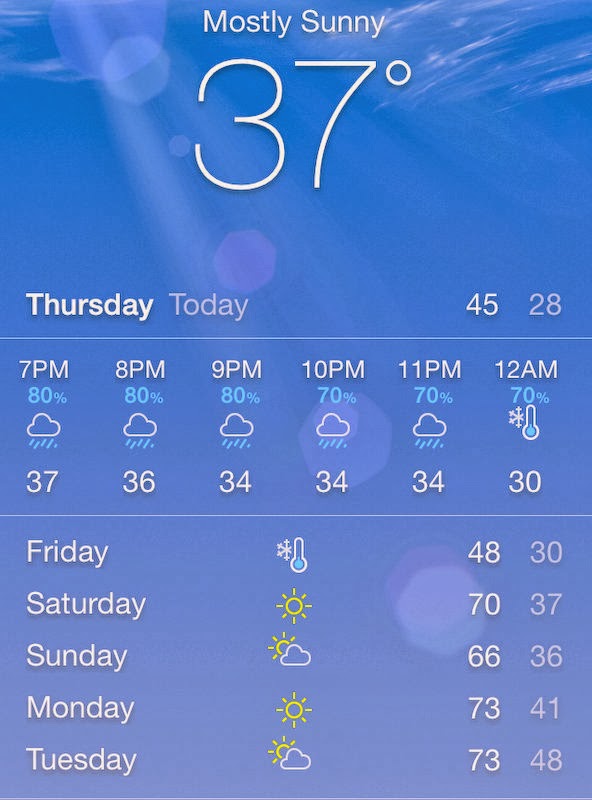The image displays a detailed weather interface with a serene blue sky background that transitions from a darker blue at the top to a lighter blue at the bottom, illuminated by a ray of light from the top left. Wisps of clouds hover at the top. 

At the top of the interface in bold white text, it reads "Mostly Sunny" with the current temperature "37°F." Directly below, "Thursday" is highlighted in a deeper white, with "Today" labeled to the right, followed by high and low temperatures "45°F" and "28°F."

The hourly forecast for the evening shows:
- 7 PM: 80% chance of rain, 37°F, accompanied by a cloud with rain icon.
- 8 PM: 80% chance of rain, 36°F.
- 9 PM: 80% chance of rain, 34°F.
- 10 PM: 70% chance of rain, 34°F.
- 11 PM: 70% chance of rain, 34°F.
- 12 AM: 70% chance of rain, 30°F.

The weekly forecast includes:
- Friday: Cold, symbolized by a blue thermometer, 48°F/30°F.
- Saturday: Sunny, 70°F/37°F.
- Sunday: Partly cloudy, 66°F/36°F.
- Monday: Sunny, 73°F/41°F.
- Tuesday: Partly cloudy, 73°F/48°F.